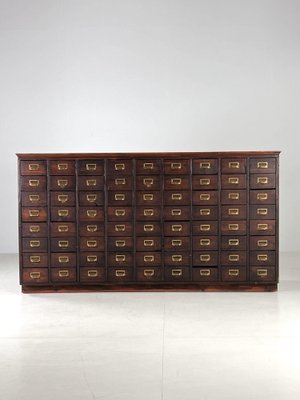The image showcases a dark brown, possibly walnut, apothecary cabinet in the style of those traditionally found in libraries. The cabinet, positioned centrally in the frame against a white backdrop and floor, comprises a grid of eighty small drawers, arranged in eight rows and nine columns. Each drawer features a central gold label holder, meant for organizing contents with small white paper labels, reminiscent of the Dewey Decimal System. All drawers are closed, and the cabinet's entirety, though not occupying a large portion of the image, is clearly visible without any obstructions or items on top.